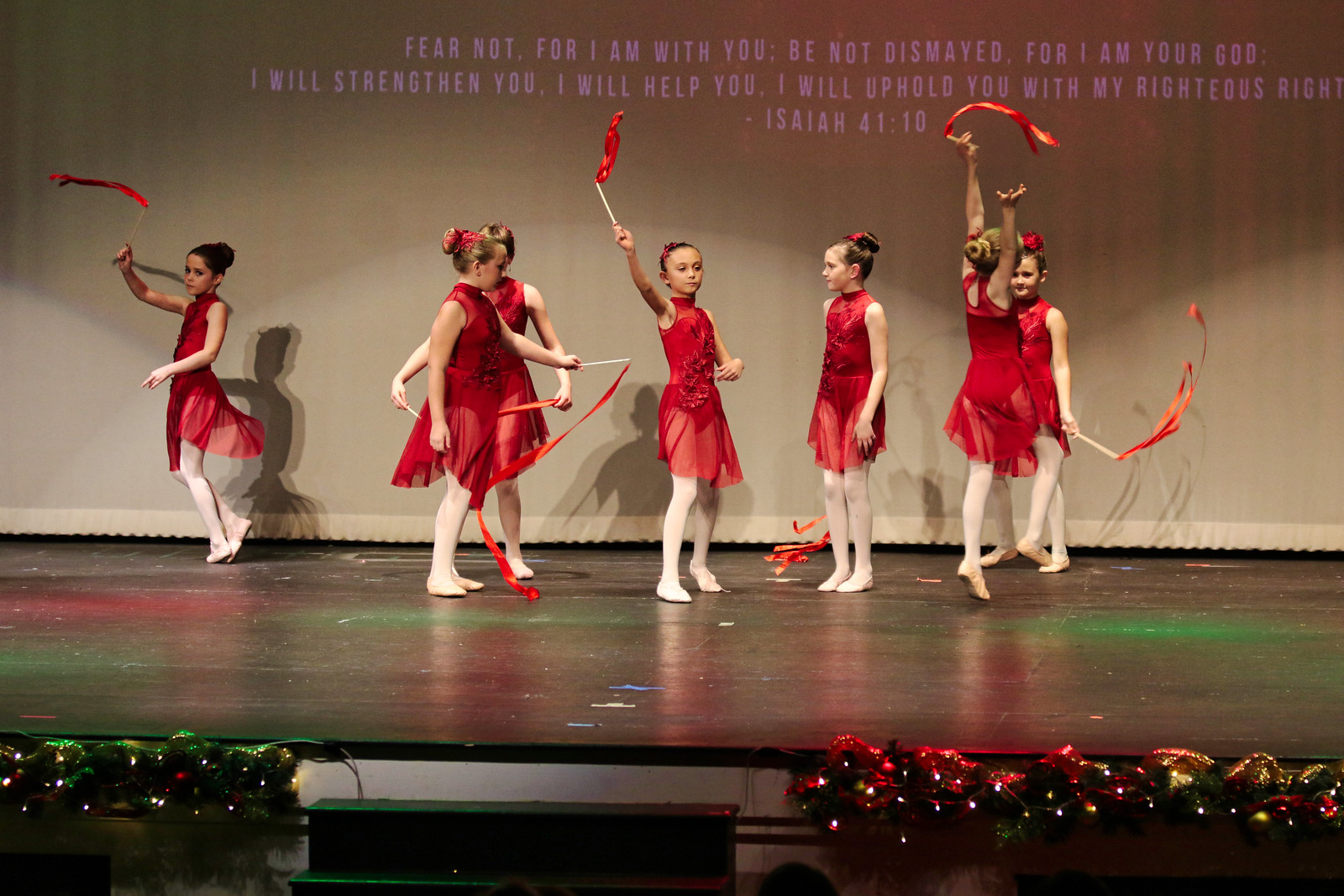The image features seven young girls, likely aged between 11 to 12 years old, performing on a stage. They are dressed in red ballet costumes with white tights and white ballerina shoes. Each girl has her hair up, adorned with red bows or ties. They are holding rods with red streamers, which they twirl as part of their ballet routine. The stage floor is a light gray-brown color, adorned with Christmas lights and ornaments along the border. The backdrop of the stage displays a projected message in white text that reads: "Fear not, for I am with you; be not dismayed, for I am your God; I will strengthen you, I will help you, I will uphold you with my righteous right hand. - Isaiah 41:10." The girls are positioned in various orientations, some facing forward, some to the side, and one with her hands raised, facing backward, adding dynamic movement to their performance. The ambient festive decor and the inspirational message create a warm and uplifting atmosphere.